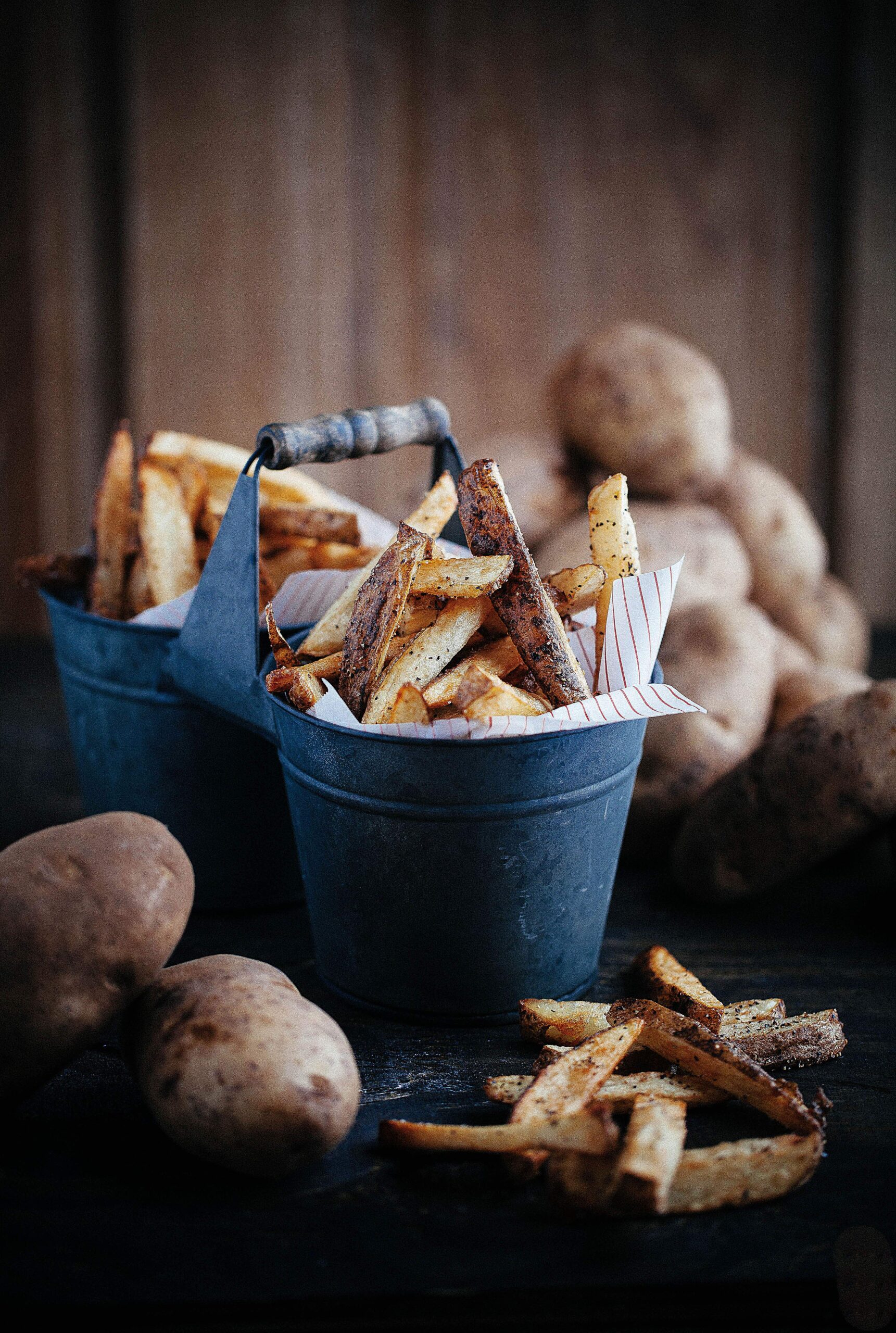The vertical rectangular image showcases two small blue buckets filled to the brim with golden-brown, skin-on French fries, seasoned with salt and pepper. These freshly made fries are spilling over onto a dark, shiny table surface. In the blurred background, a rustic wooden wall sets the stage, stacked with whole, unpeeled potatoes. Additional unprocessed potatoes flank the buckets, hinting at the homemade origin of the fries. The blue buckets contain paper liners, and between them, there is a notable wooden handle for easy carrying. The color palette features tones of brown, blue, and various shades of tan, evoking a cozy, rustic atmosphere. This appetizing scene would be perfect for a recipe website, showcasing the process and final product of homemade, skin-on French fries.